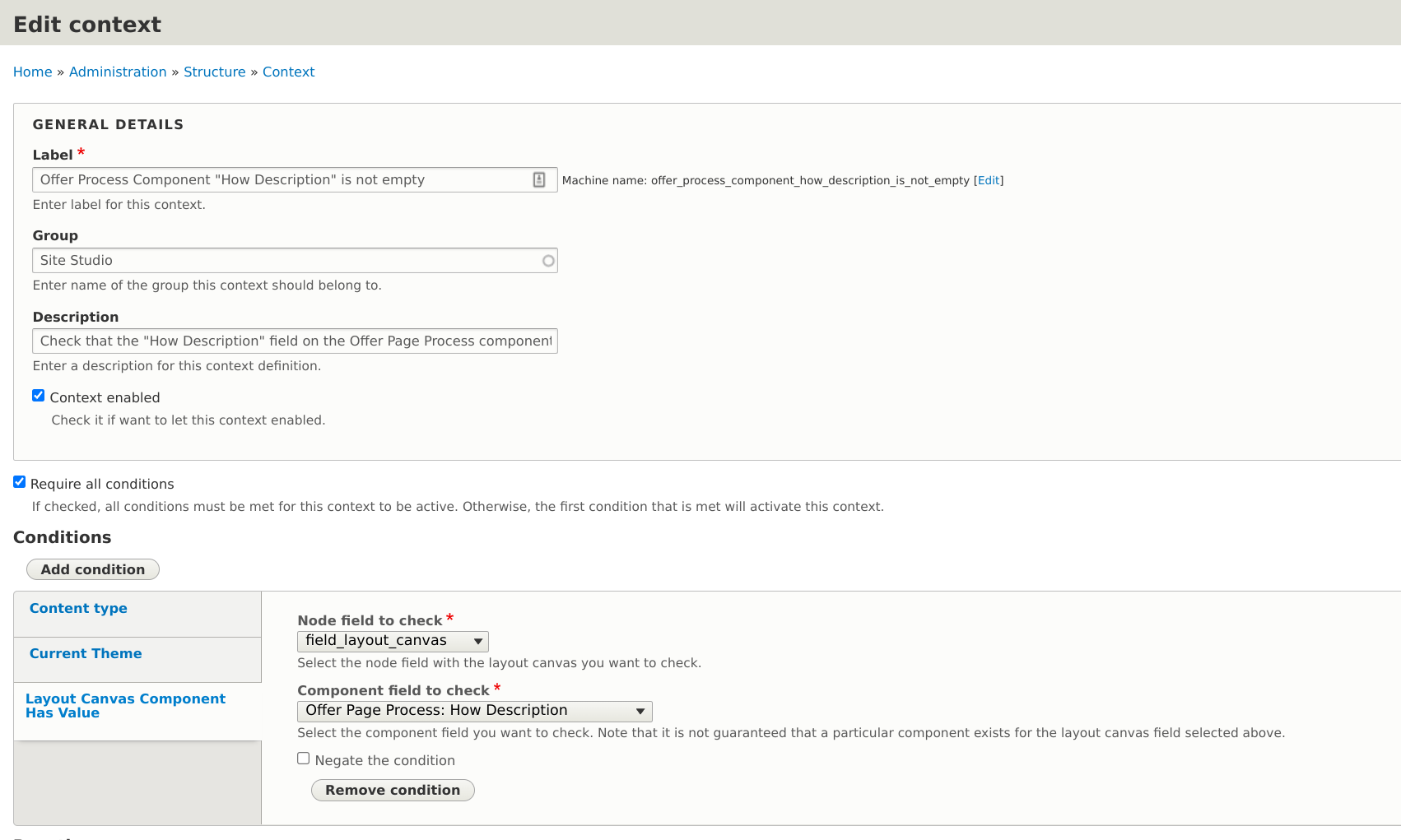A screenshot displaying a detailed dashboard interface of a software application is shown. The top bar, labeled "Edit Context," is dark gray and contains options such as "Home," "Administration," "Structure," "Context," and "General Details" arranged sequentially. Below, there are various fields and labels, including "Label Field," "Group Field," and "Description Field." 

Several options are enabled with blue checkmarks: "Context Enabled," "Acquire All Conditions," and a bold text labeled "Conditions." Other categories highlighted in blue include "Content Type," "Content Theme," "Layout," "Canvas Component," "Max Value," and "Node Field." 

A dropdown menu is marked with a red asterisk, indicating it is mandatory, and is labeled with black text that reads: "Select the node field with the layout canvas you want to check." An adjacent field, which is somewhat unreadable, contains the text "Remove Condition."

The background is shaded in varying tones of gray, with the top bar being the darkest. The overall composition of the screenshot showcases the software's interface for editing context parameters and conditions.